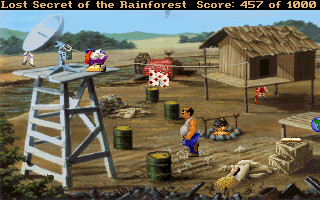This image is a detailed screenshot from a video game titled "Lost Secret of the Rainforest," as displayed on the black bar at the top of the screen with a score of 457 out of 1000. The scene depicted appears to be a rustic, farm-like outdoor setting dominated by an earthy dirt surface. Central to the scene is a small, elevated wooden barn or shack on stilts with a thatched roof, described as brown in color and resembling a rustic hut. Suspended overhead is a wire clothing line holding red and white shorts or underwear. Nearby, an outdoor fire pit encircled by stones has a black pot hanging above it. 

There is a tall, rickety wooden tower painted white or silver that supports a small satellite dish pointed to the left, with cables extending from it toward the barn. The tower also includes stairs and a red and yellow object perched on it. Scattered around the area are several green-colored oil drums, boxes, and crates of various materials. Vegetation such as trees, brush, and rolling hills can be seen in the background of the scene.

In the foreground, a cartoonish man with blue pants, a white shirt, dark hair, and a noticeable beer belly stands prominently. Additionally, off to the side, there appears to be a young girl, viewed from the back, near the stilted house.